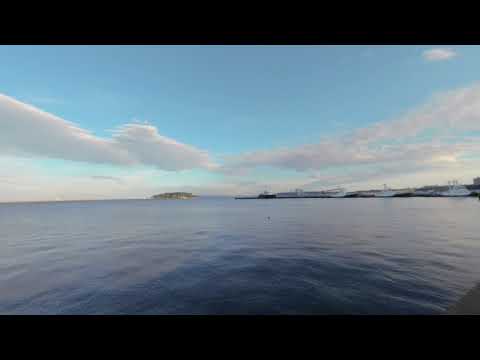This blurry, rectangular photograph depicts a serene ocean scene taken from the vantage point of land. In the center of the image, amid a mostly blue expanse of water, there is a hint of a pier with boats docked alongside it. Towards the left of the pier, an indistinct, green and yellow form suggests a small distant island rather than a nearby vessel. The sky above is dotted with clouds that curve around a central clearing, revealing a clear blue sky above the horizon line. The water below transitions from light blue on the sides to a deep, dark blue near the bottom of the image, enhancing the depth and calmness of the seascape.